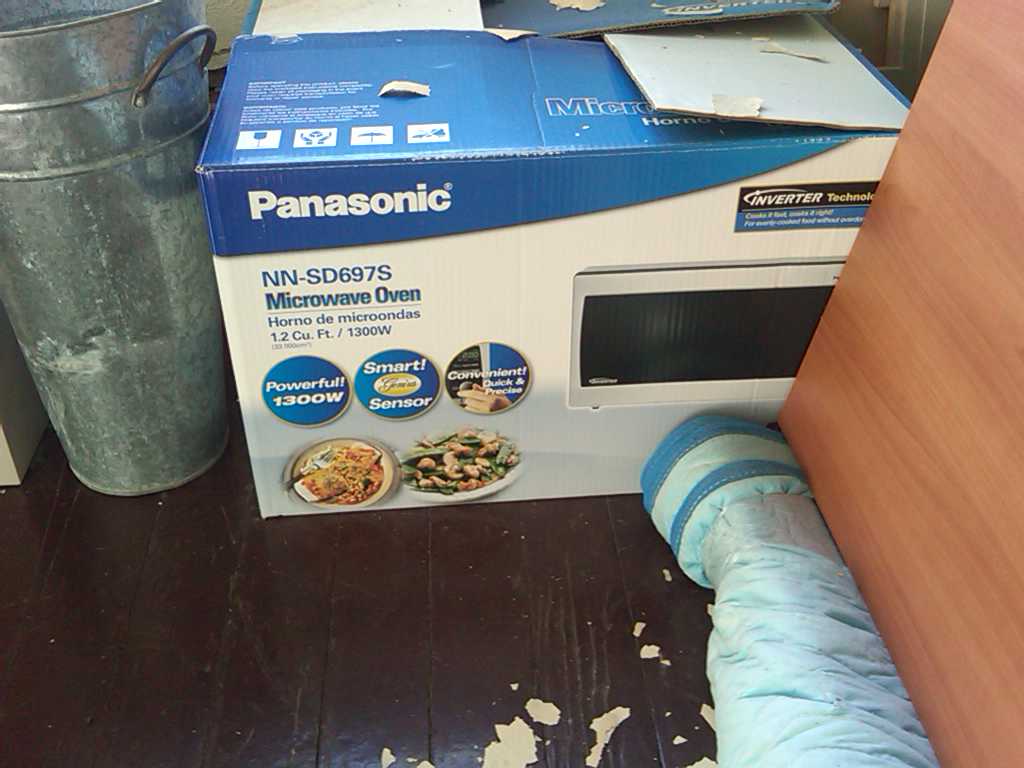The image depicts a realistic indoor scene focused on a dark hardwood floor, which exhibits some wear and tear such as flakes or cracks. Dominating the center of the image is a partially opened cardboard box, primarily white with a blue top, featuring branding and product details. The box is labeled "Panasonic" in white lettering on the blue section and "NN-SD697S Microwave Oven" in blue letters on the white part. Additionally, the box displays features like "1.2 cubic feet," "Powerful 1300 Watt Smart Sensor," and "Convenient" in blue circles. 

In the upper left corner of the image, there are one or two weathered, silver galvanized metal buckets or pails, suggesting signs of frequent use. To the right of the box and partially cut off by the frame is a tall, light-colored piece of wood, which could be a wall or a piece of furniture. Beneath this wooden element lies a rolled-up light blue blanket or table covering. The microwave box also shows an image of the appliance, with specific details like a white outer edge and a black screen area. Overall, the scene is a blend of utilitarian objects and a setting that hints at both functionality and wear.